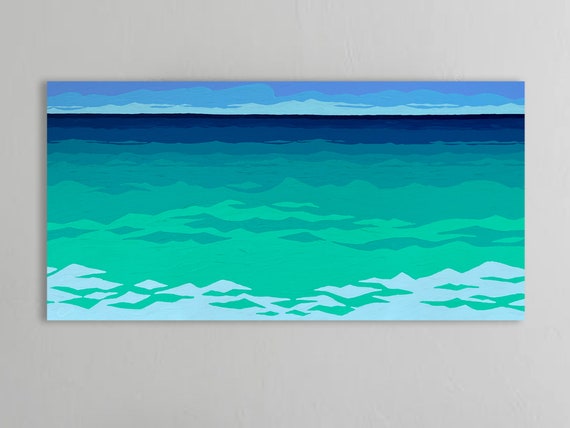This is a unique and detailed watercolor painting of an ocean, prominently displayed on an off-white or light gray gallery wall. The painting is in a long rectangular format and features a stylized, abstract depiction of a seascape, rather than an accurate rendering. The water exhibits a gradation of colors: from an aqua green close up, transitioning into various shades of teal, deepening to blues, and eventually to almost black as it recedes into the distance. Gentle, rolling waves and ripples suggest the motion of the water, which appears to be neither completely calm nor highly turbulent, embodying a tranquil daytime scene. The horizon showcases a medium to deep blue sky with wispy clouds, creating a subtle distinction between the sea and the sky. Interspersed among the waves are white frothy peaks, hinting at the waves' crests. Overall, the painting is minimalist yet expressive, capturing the serene but dynamic essence of an ocean view.